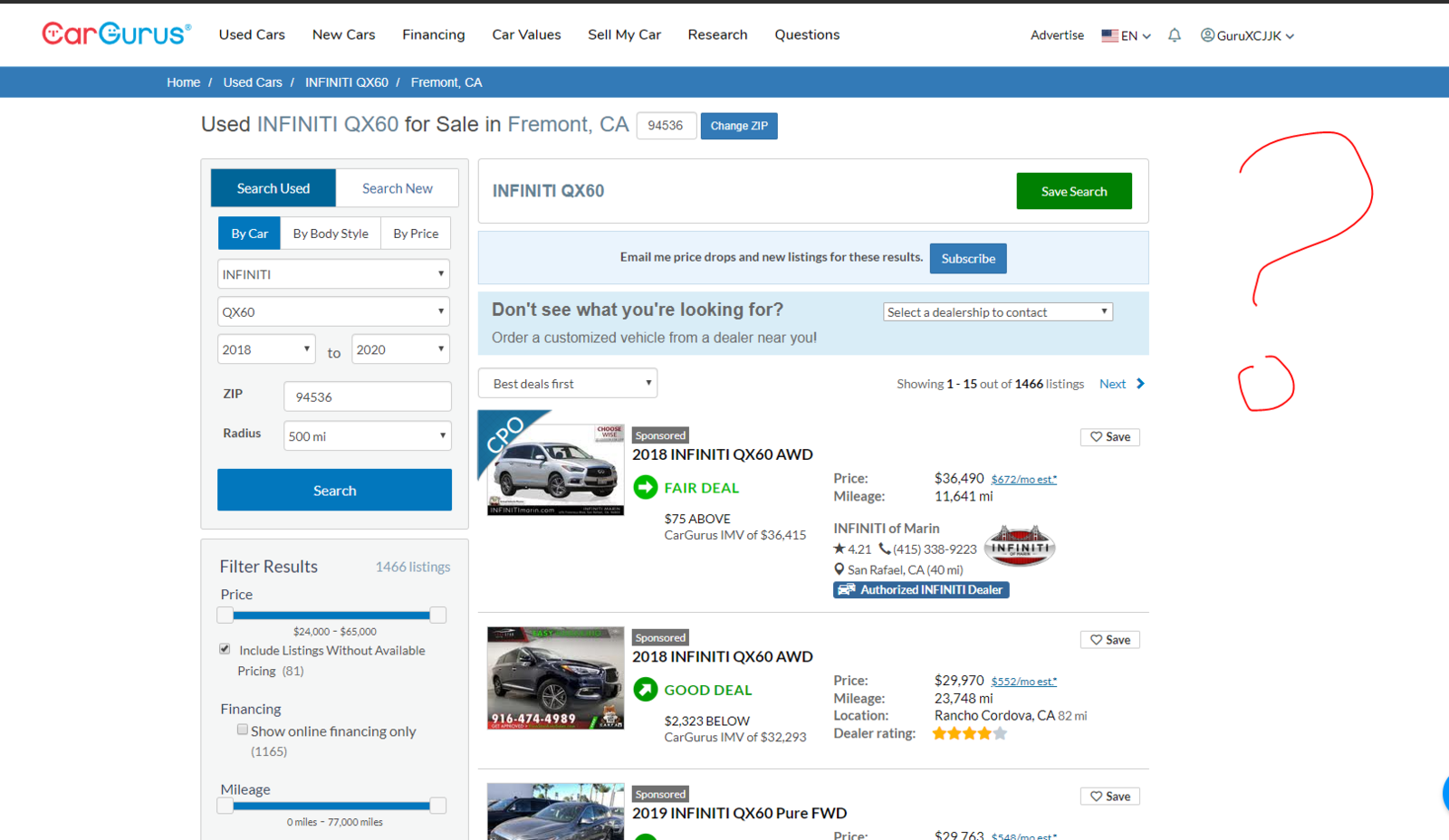In this screenshot, the user interface features a predominantly white background. At the upper left-hand corner, the logo "car gurus" is displayed, with "car" in red and "gurus" in bright blue. Adjacent to the logo are several categories listed horizontally: "used cars," "new cars," "financing," "car values," "sell my car," "research," and "questions." 

To the right of these categories, there's an "advertise" option followed by an icon of the American flag, a notification bell, and a username that appears to be "Gen X C JJK." Below the navigation bar, a red strip houses more options like "home," "used cars," "infinity," an unreadable item, "fireman," and "Cal, CA," all in white text against the blue background of the strip.

The layout below this navigation includes a search section on the left side. Here, users can filter searches by various criteria with white input boxes and dropdown menus; options include searching by "body style," "price," and other specifications. There’s a section titled "filter results," allowing adjustments such as price and mileage to be tailored to individual needs.

Towards the central area, there’s a headline for an "Infinity QX60" with a green button labeled "start search" prominently placed next to it. Beneath this, a blue section appears with instructions to subscribe via a blue button labeled "subscribe." This is followed by another message that prompts users who can’t find what they are looking for to "order a customized vehicle from a dealer near you," featuring a search box to select dealerships for contact.

In the bottom section, options like "best deals first" with a search box are present. The interface showcases three car listings with labels such as "fair deal," "good deal" set within green, rounded arrows. Each car’s listing provides detailed information including images, prices, mileage, dealer ratings, and other specifics.

To the far right, adjacent to the car listings, a red question mark is handwritten in a wavy style using online pen ink. The dot of the question mark is encircled. This hand-drawn addition seems to be a personal annotation added to the screenshot, potentially to highlight or query some part of the interface.